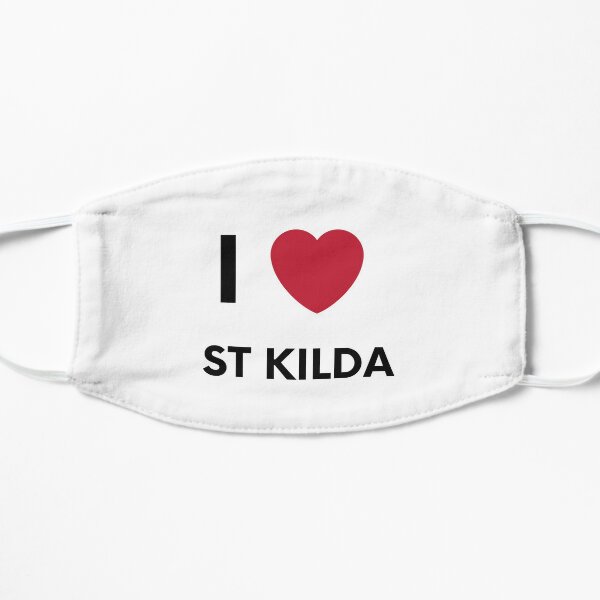The image features a plain white cloth face mask, typically worn over the nose and mouth during the COVID-19 pandemic. The mask is prominently displayed lying flat on a solid white surface, with soft shadows indicating where its edges are slightly raised. The focal point of the mask is a bold graphic in the center, which reads "I ❤️ Saint Kilda." The text is printed in black, with the heart symbol rendered in a vibrant red. The layout includes a large letter "I" to the left of the heart, and the words "St Kilda" are positioned below, in smaller black font. The simplicity of the backdrop enhances the visibility of the mask’s design.